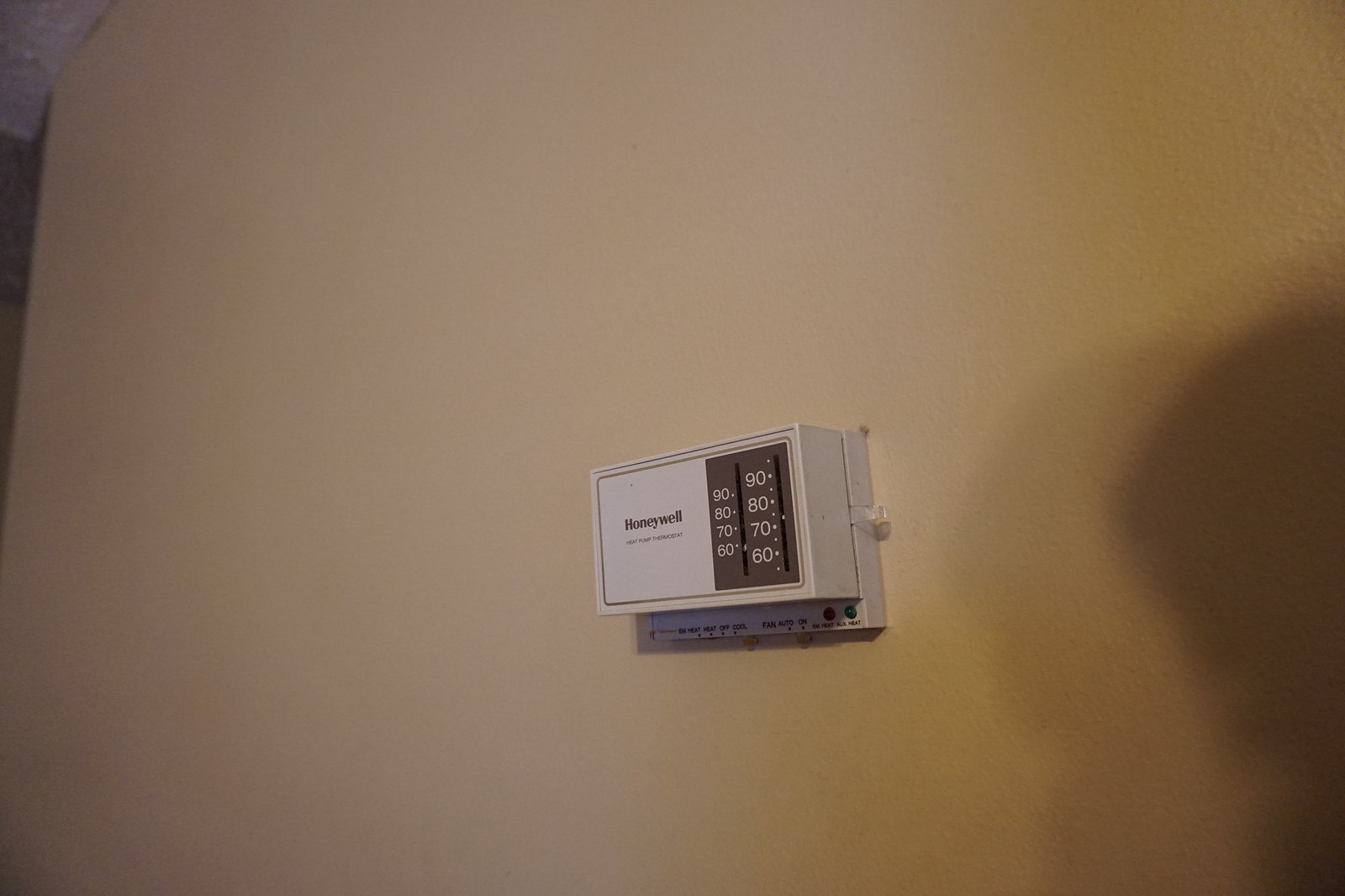The image depicts a beige-colored wall featuring a prominently mounted thermostat designed to control the air conditioning units in the home. The thermostat, encased in a rectangular tan and deeper brown plastic casing, prominently displays the brand name "Honeywell" on its face. The temperature gauge on the thermostat is marked with numbers ranging from 60 to 90 degrees Fahrenheit. A noticeable plastic handle protrudes from the right side of the device, which is used to adjust the temperature settings, ensuring the desired indoor climate is maintained effectively.